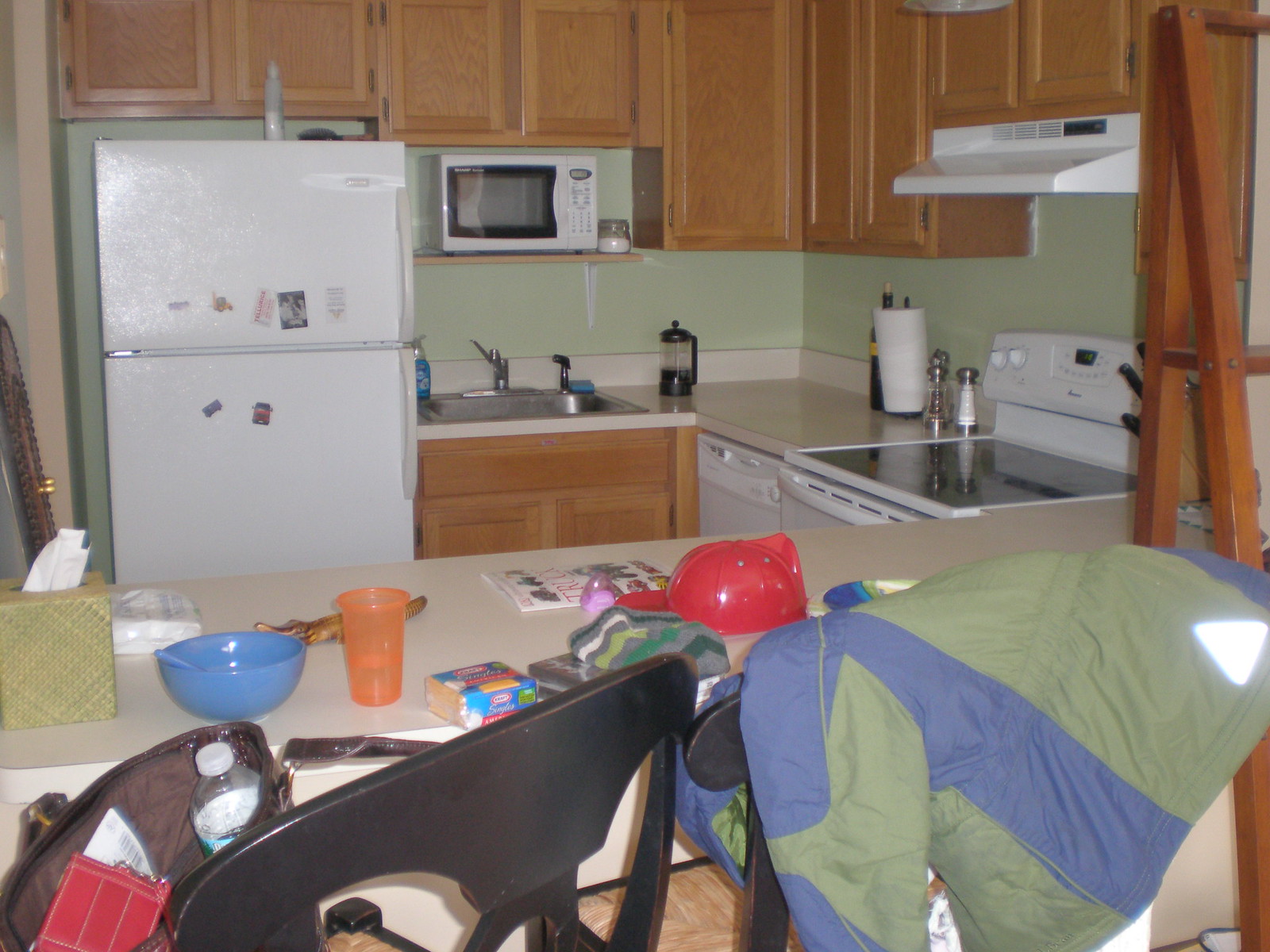In this cozy kitchen, there are rich brown cabinets that contrast beautifully with the white appliances, including a stove and hood, and a microwave. A limited amount of counter space leads to a single sink. To the left of the sink, a white refrigerator stands tall. In the foreground, there's a counter lined with dark brown bar stools that have tall backs, creating a perfect spot for casual dining. The counter is cluttered with various items such as a blue bowl, an orange glass, an open pack of cheese, a red helmet, a magazine, and a box of tissues situated on the far left. Draped over the backs of the bar stools are a green and blue jacket and a dark brown purse rests on one of the seats. The kitchen area is a medley of neutral tones like black, tan, and dark brown, accented with pops of silver, blue, orange, and red from the assorted items atop the counter. It depicts a lived-in home with a warm and personal touch.